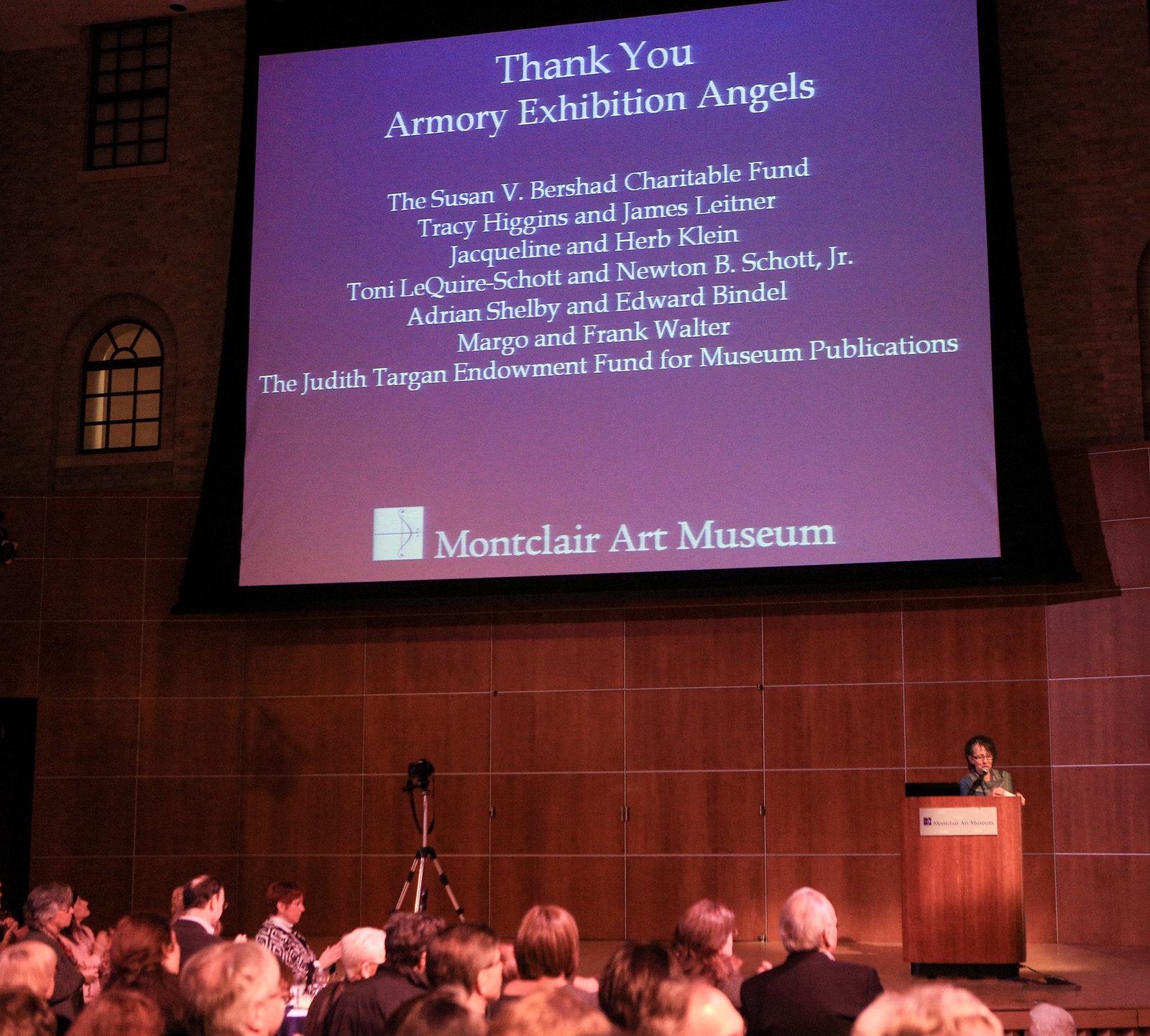The image depicts a scene from a lecture or seminar held in a large room at the Montclair Art Museum. A woman with dark hair and glasses stands behind a wooden podium bearing the museum's name. The backdrop features a large projection screen with a purplish background displaying white text. The text reads, "Thank you Armory Exhibition Angels," followed by a list of donors: the Susan B. Bouchard Charitable Fund, Tracy Higgins and James Leitner, Jacqueline and Herb Kline, Tony Laquire Schott and Newton B. Schott Jr., Adrienne Shelby and Edward Bindel, Margo and Frank Walter, and the Judith Targan Endowment Fund for Museum Publications. Below this list, "Montclair Art Museum" is also mentioned. The audience sits facing the presenter, with about 20 individuals visible from behind. Additionally, there is a camera on a tripod situated near the stage, and two windows with distinct shapes—one rectangular with bars and one rounded—are visible to the left of the screen.